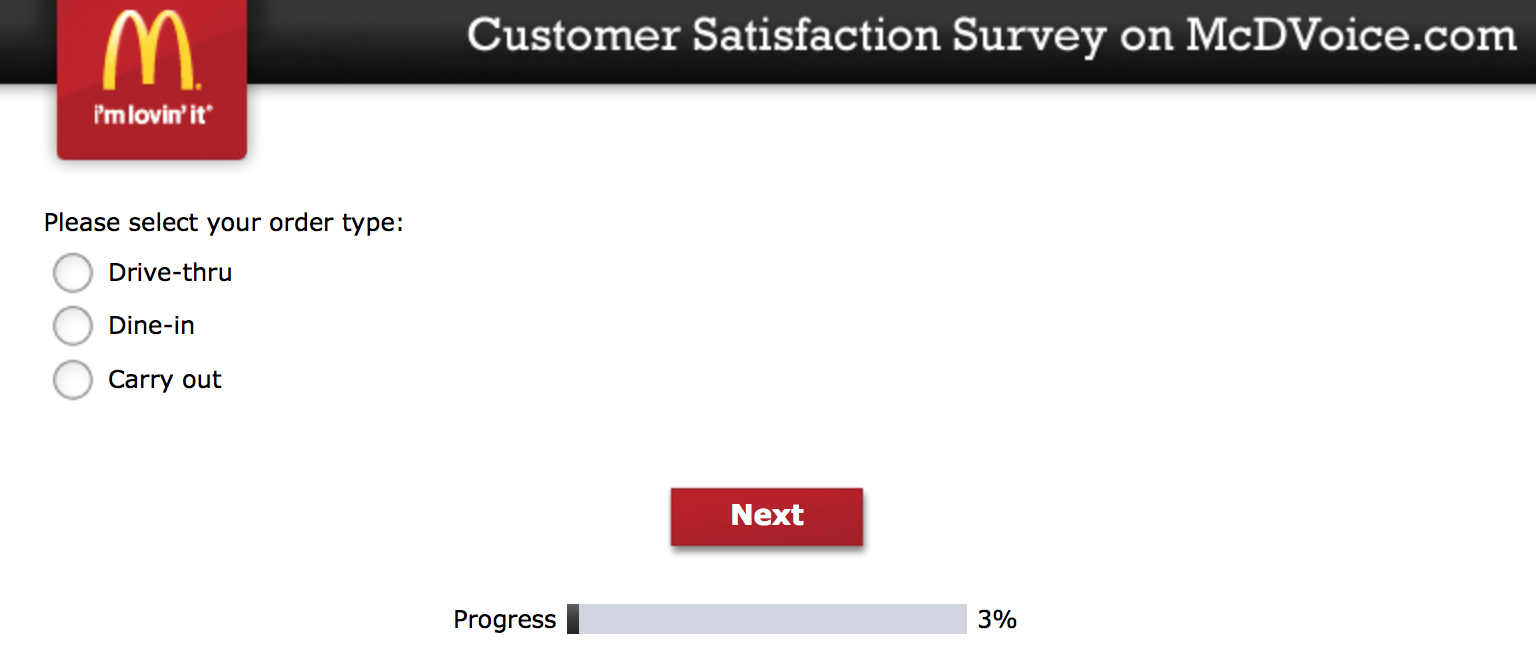The image depicts a webpage or app interface for McDonald's, distinguishable by the McDonald's logo at the top. The header features a black border running across the top, with a red square situated on the left side. Within this red square, the iconic McDonald's 'M', also known as the Golden Arches, is prominently displayed in yellow. Directly beneath the logo, the slogan "I'm Lovin' It" appears in white text, with an apostrophe replacing the "g" in "Loving."

To the right of the logo, the header contains a message in white text: "Customer Satisfaction Survey on MCDVoice.com." Below this header, aligned to the left and under the logo and slogan, the text "Please Select Your Order Type…" is displayed in black, with three unselected circular options below it. The options are labeled in black text as "Drive-Thru," "Dine-In," and "Carry Out." Adjacent to these options, a red rectangular button at the bottom center of the screen features the word "Next" in white text.

At the bottom of the interface, a progress bar is visible, indicating "Progress" on the left side and showing that the progress is at 3%, with this percentage displayed on the right side of a gray rectangular segment.